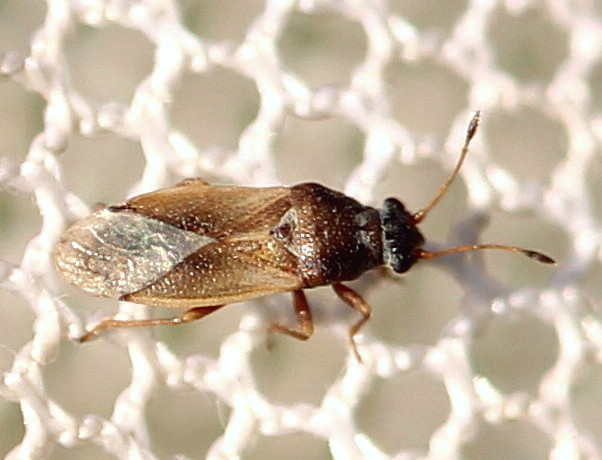In the highly detailed close-up shot, the insect's striking features are vividly magnified. The insect, predominantly black, brown, and white, is oriented facing right within the frame. It boasts a triangular-shaped head, adorned with two bulbous eyes positioned laterally, and dual antennae protrude centrally. The brown, multi-directional antennae culminate in darker brown bulbs. Its body is broad and tinged in brown with sporadic white spots, leading to its folded wings. These wings are cloaked in a transparent brown protective layer and exhibit distinct white veins. Only three of the insect's six legs are conspicuous, all situated towards the lower part of the image, while the other three remain obscured by the sideways perspective. The insect is perched on a net-like material composed of interwoven white strands, set against a gray background adorned with white, rope-like circular patterns.